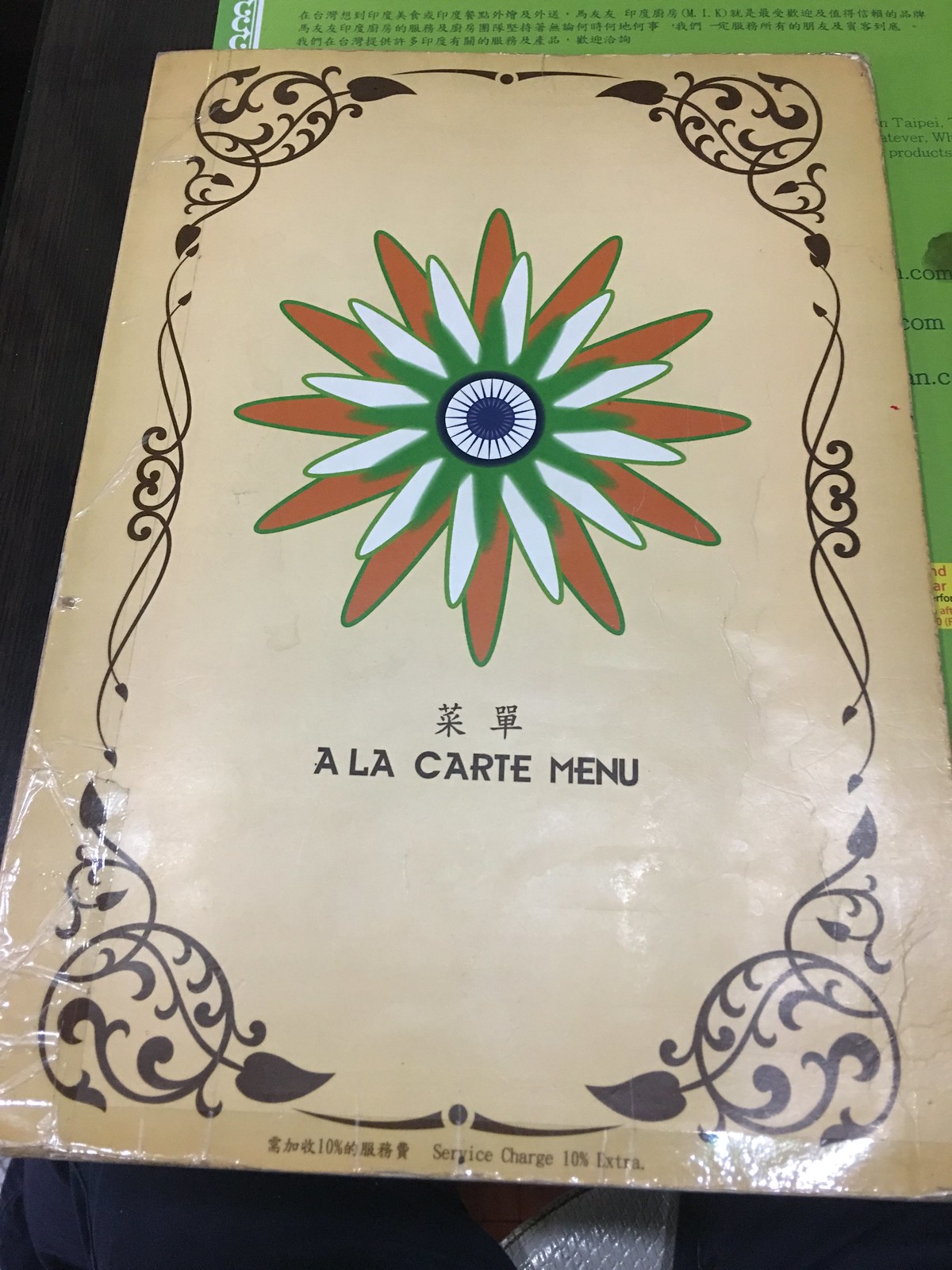The image features an elegant menu with a beige background. At its center is an intricate, eye-catching design resembling both a sun and an eye, created using black and white lines that radiate outward. This central motif is encircled by layers of decorative elements: first, green, star-like and flower-like leaves, followed by white, pointed leaves arranged in a larger pattern. Beyond this is an expansive border of orange leaves with a green outline, all framed by a delicate, black floral border that provides ample space around the edges.

Underneath the central flower-like image, Asian characters are prominently displayed alongside the text "A La Carte Menu." At the very bottom center, additional Asian writing can be found, along with a note indicating a service charge of 10% extra. A green piece of paper is partially visible behind the menu, adding a subtle pop of color to the overall composition.